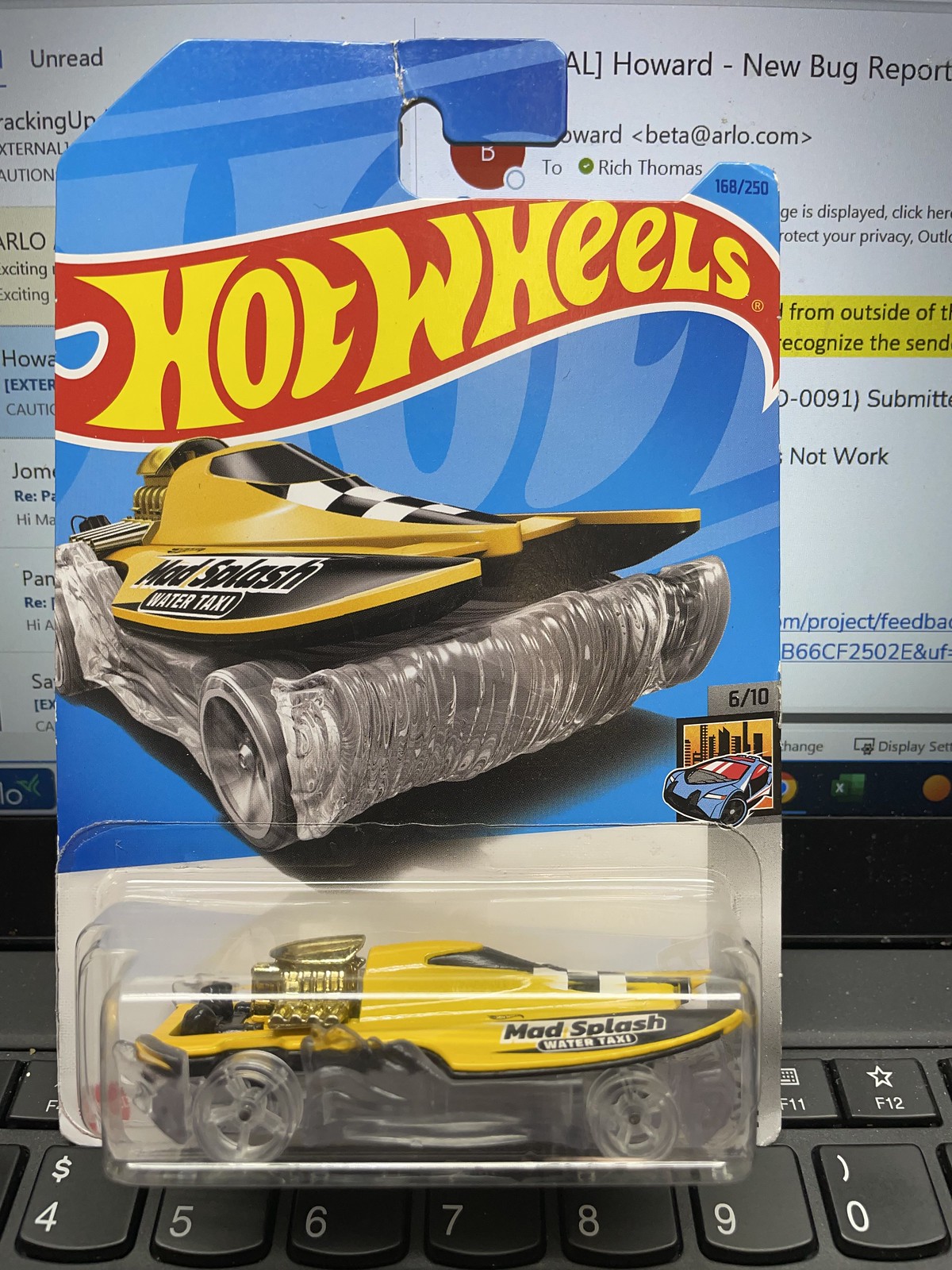The photograph captures a mint-in-package Hot Wheels car titled "Mad Splash," prominently displayed on the keyboard of a laptop. The Hot Wheels packaging features a vibrant blue background with a red banner that has "Hot Wheels" written in bold yellow text. The car, designed to resemble a sporty water taxi, flaunts a striking yellow top adorned with black and white checkered flags and appears to be splashing through water, indicated by the water-themed details around its tires. The car's packaging indicates it is a collectible item, numbered 6 out of 10. The Hot Wheels car remains unopened in its pristine packaging, positioned over the laptop's numeric keys 4 through 9. In the background, the laptop screen shows an open email application, partially displaying a message titled "New Bug Report Beta" from Howard at Arlo.com, addressed to Rich Thomas, with highlighted areas in blue and yellow for emphasis.